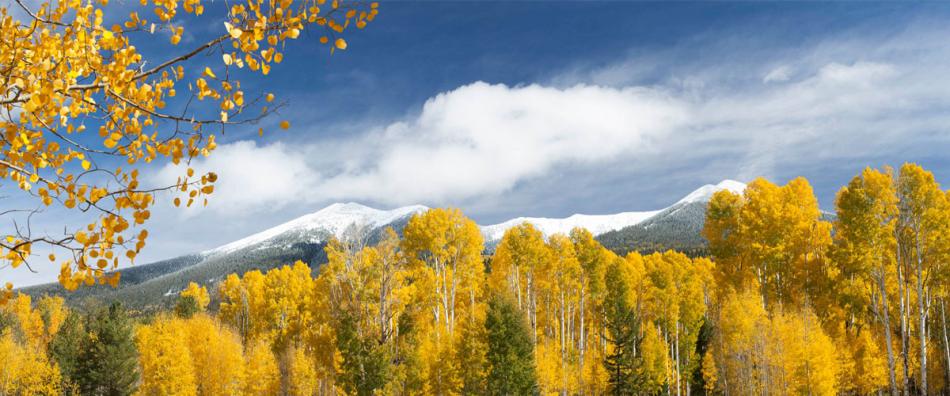This captivating outdoor image showcases a serene autumn forest with a rich tapestry of colors and details. In the foreground, a diverse array of tall trees display vibrant golden leaves, interspersed with some still holding onto their green foliage. These trees create a beautiful gradient from left to right, with one particularly prominent green tree on the far left. A closer inspection reveals the trunks of these trees, pristine white against the autumn hues, adding texture to the landscape. Intriguingly, a branch with round yellow leaves, reminiscent of ginkgo leaves, extends from the left third of the image.

In the background, majestic mountains capped with a pristine layer of snow rise in the distance, adding a dramatic contrast to the vivid forest below. Above, a dynamic sky transitions between a rich blue and clusters of puffy white clouds, which seem to flow gently from right to left across the scene.

The interplay of colors – from the bright yellows and greens of the foliage to the crisp whites of the tree trunks and snow-capped peaks, set against the deep blue sky – captures the essence of a tranquil autumn day in nature’s embrace. The overall imagery exudes a peaceful, almost ethereal beauty, making it a serene and picturesque landscape.